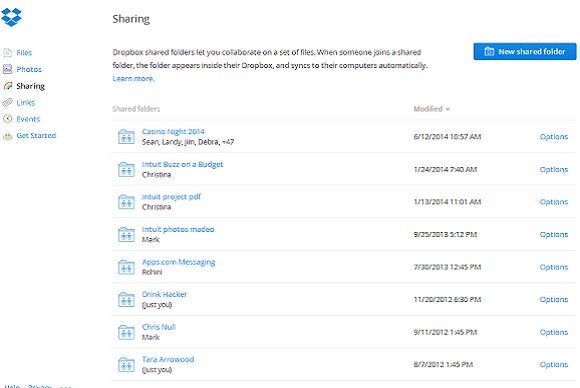The image is a detailed screen capture from a desktop, showcasing the Dropbox application's interface. Dominating the upper left side of the image is the familiar blue Dropbox logo. The main screen features a clean, white background with the heading "Sharing" prominently displayed at the top in bold, black text. Just below this heading, a smaller black text describes the purpose of shared folders in Dropbox: "Dropbox shared folders let you collaborate on a set of files."

On the upper right side of the screen, a blue rectangular button stands out with white text that reads, "New shared folder." This button is meant for initiating the creation of new shared folders. Directly below this section, there are multiple rows of folders aligned to the left. Each folder is represented by an icon depicting two people, indicative of shared access.

Each row contains crucial information about the folders, starting with the folder name and followed by the list of collaborators. At the top row, the folder is named "Casino Night 2014." Beneath this folder name, in smaller black text, are the names of the individuals who have access to this shared folder. This layout exemplifies how Dropbox organizes and displays shared content, making it easy to identify and manage collaborative projects.